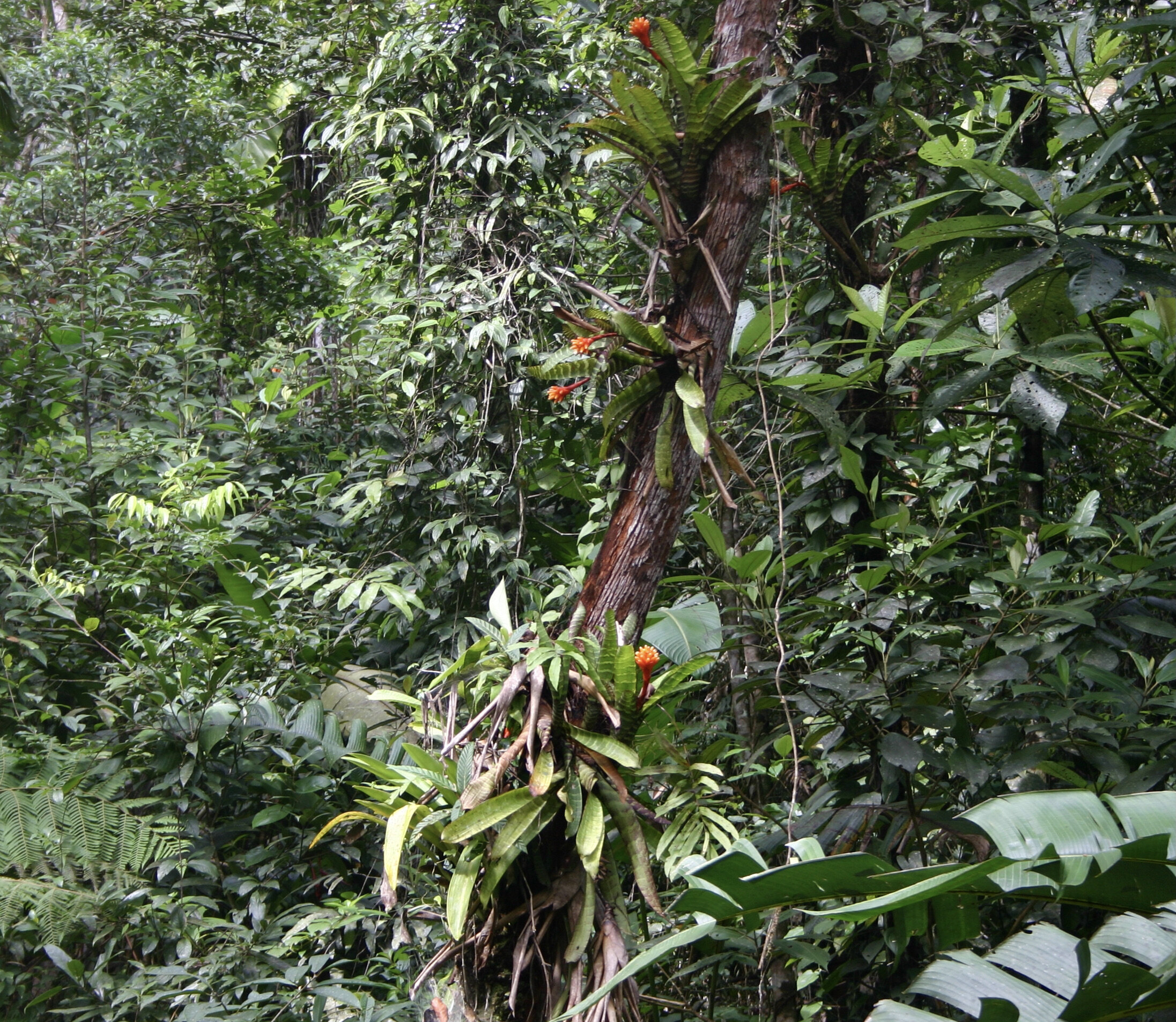The image captures a lush and densely overgrown outdoor scene, possibly a forest or jungle, bathed in daylight. Dominating the center is a tall, slender tree trunk covered in numerous broad green leaves sprouting from the ground up, each leaf brimming with vibrant life. Scattered among these leaves are striking orange flowers, adding a pop of color against the green foliage. The backdrop is a verdant expanse of various plants, including ferns and bushes, with large leaves extending into the frame. The scene is so densely packed with plant life that neither the sky nor the ground is visible, emphasizing the vitality and overgrown nature of the area. Sunlight filters through, creating bright spots on the leaves, enhancing the vivid greens and oranges. The overall impression is one of a thriving, untamed natural environment.